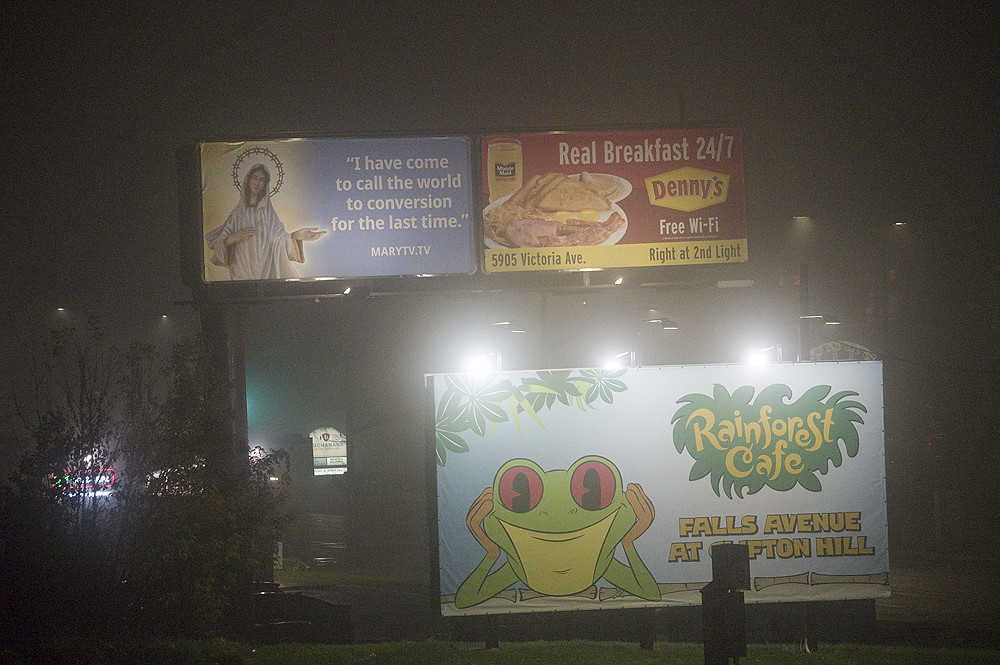A nighttime street scene unfolds in this photograph, which is wider than it is tall. The image is taken from a road, illuminated by several street lights in the background, casting a soft glow that hints at moisture in the air. The main subjects of the photo are eye-catching billboards that dominate the urban landscape.

In the bottom right corner, a large, vibrant billboard advertises the Rainforest Café, located at Falls Avenue and Clifton Hill. The advertisement features a friendly, animated frog facing the viewer, set against a lush, leafy backdrop with a clear blue sky peeking through.

Towards the top left of the image, a larger but more distant billboard captures attention with its dual messages. One part of the sign declares, "I have come to call the world to conversation one last time," and directs viewers to MaryTV.tv. This segment of the billboard includes an image of what appears to be either the Virgin Mary or a Christ-like figure. Adjacent to this, the second part of the billboard is an advertisement for Denny's, promoting real breakfast available 24/7 with free Wi-Fi at 5905 Victoria Avenue, right at the second light. The Denny's ad features a bold red background with yellow accents, showcasing delicious bacon and eggs.

The overall ambiance of the photograph is enhanced by the soft, diffused lighting provided by the street lamps, lending the scene a subtle neon flair and enveloping it in a cozy, nocturnal atmosphere.